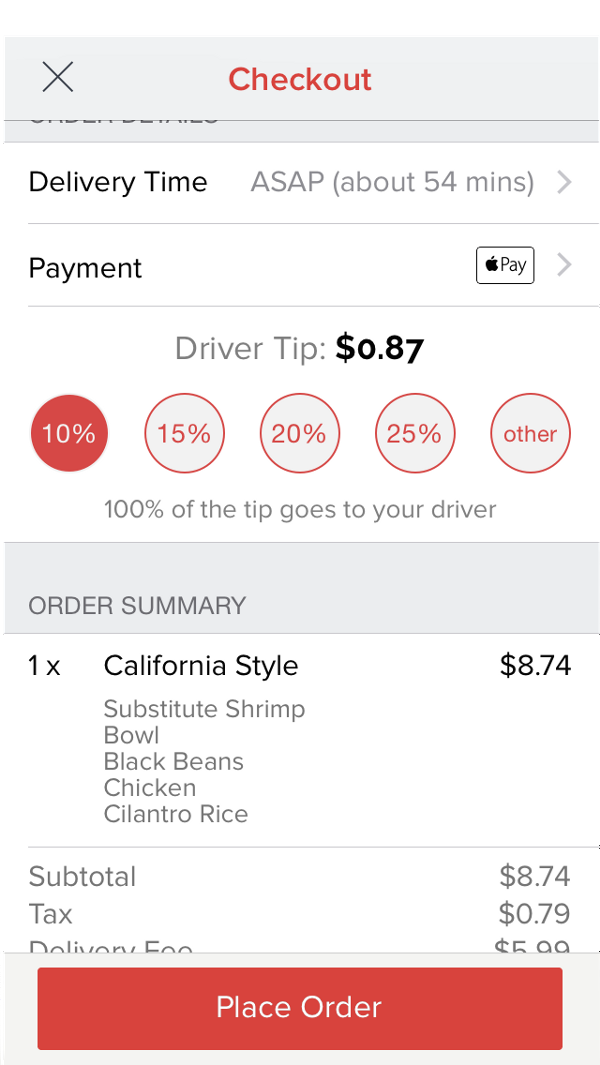The image showcases a detailed breakdown of an order summary and payment information for a food delivery service. 

At the top, written in orange text, is the phrase "Check Out," with a grey "X" icon to the left indicating the option to close the window. Directly below, grey text reads "Delivery Time, ASAP, about 54 minutes."

Continuing downward, information on the selected payment method is provided: "Payment" displaying an Apple Pay logo with the text in black. 

Below the payment details is the "Driver Tip" section, indicating a tip amount of $0.87. Here, there are five orange circles representing different tipping percentages. The circles are labeled 10%, 15%, 20%, 25%, and "Add." The first circle, marked 10%, is highlighted in orange to show it is the selected tip amount. Accompanying this section is the statement, "100% of the tips go to the driver."

Next, the "Order Summary" outlines the specifics of the order: 
- 1x California Style Bowl ($8.74) including substitute shrimp, black beans, chicken, and cilantro rice.

The order subtotal is listed as $8.74, with an additional tax of $0.79 and a delivery fee of $5.99. 

At the bottom of the image is an orange button labeled "Place Order," inviting the user to complete their purchase.